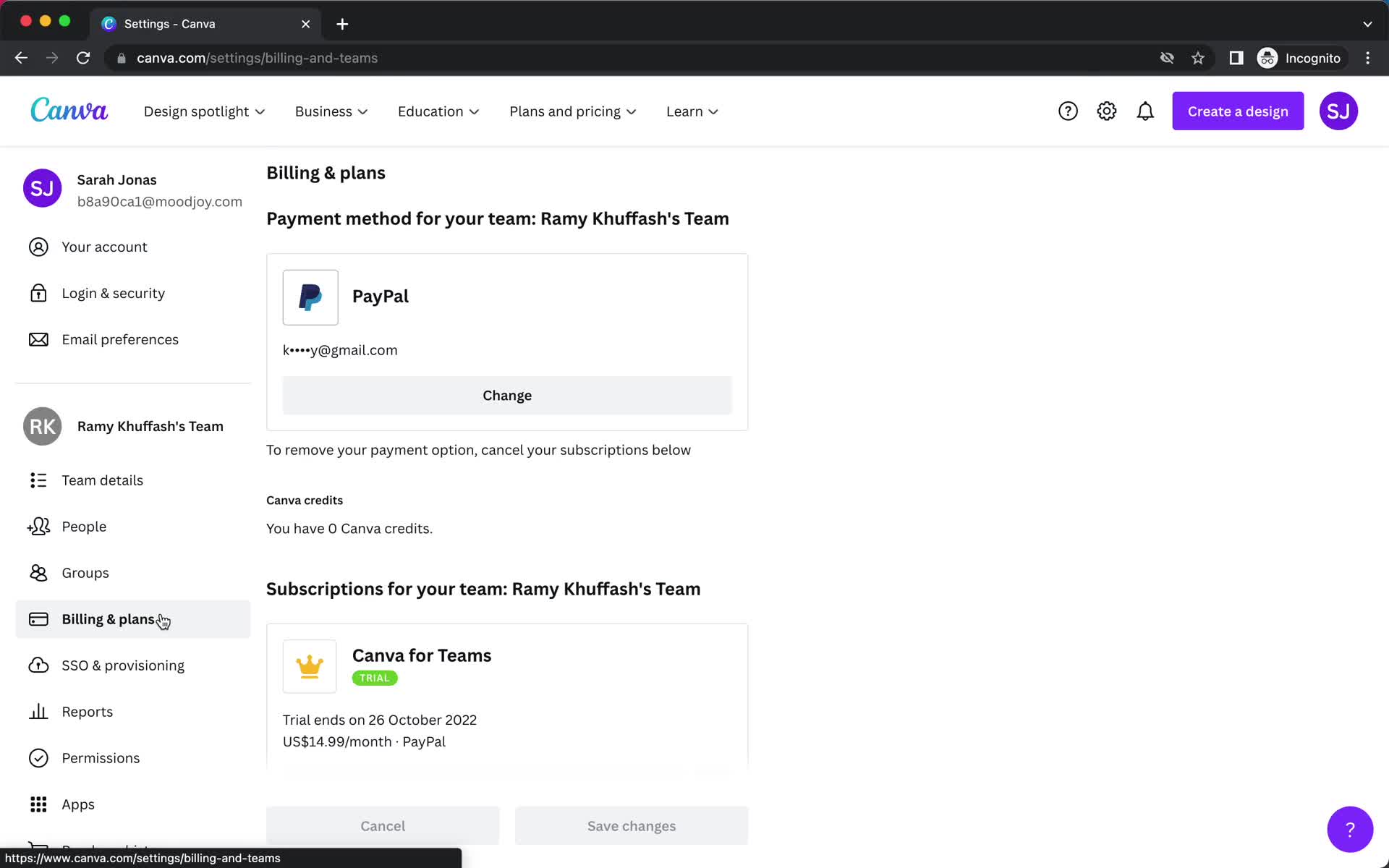The top portion of the image features a black toolbar with three circles in the top left corner: a red circle, a yellow circle, and a green circle. Adjacent to these is a tab represented by a blue-to-light-blue-to-purple circle. Beneath this is a white, dashed canvas with a white X in the center. Accompanying it are navigational arrows: a white arrow pointing to the left, a gray arrow pointing to the right, and a refresh icon represented by a circular arrow.

The main content displayed is a web browser window addressed at "whitecamera.com/billing-ante-teams". Within the browser, there's an incognito mode indicator: a white circle featuring a black head with black glasses and a white label reading "incognito". On the left side of the browser window, there are navigation options in black text: Design, Spotlight, Business, Education, Plans & Pricing, and Learn.

The webpage shows a section titled "Billing and Plans", detailing payment information for a team named "Run Me Too Fast". The team’s current payment method is listed as PayPal, identified by the partially obscured email "k*****y@gmail.com". Next to it, there's an option to "change" the payment method or cancel the subscription. 

Additionally, it specifies that the team has "0 camera credits" remaining. Under the subscription details, it notes that the team’s "Camera for Teams" trial, highlighted in a green oval with "TRIAL" in white text, is set to end on 26 October 2022, after which the team will be billed $14.99 per month via PayPal.